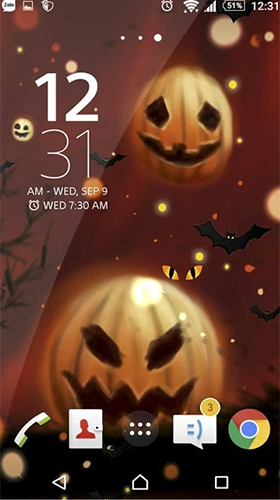This screenshot captures a detailed Halloween-themed phone background, dominated by a spooky and sinister visual motif. The background gradient transitions from a deep burgundy red at the top to a pitch-black at the bottom. In the top right corner, a small orange circle is visible, partially obscure by a witch's silhouette. Below, a prominent pumpkin with black eyes and mouth appears, accompanied by a bat to its left and another bat slightly down to the right.

At the very bottom, a larger pumpkin with evil, jagged teeth and crooked eyes menacingly grins, set against a backdrop with several smaller bats scattered around. 

In the top-left corner, a black square displays "Zolt" in white text, flanked by basic phone status icons: picture, shield, time (12:31), battery level (51%), full internet signal, full Wi-Fi signal, and an active alarm icon. Centrally below these status icons is a trio of dots—a small one on the left, a small one on the right, and a larger one in the middle.

Continuing down the screen, the date display shows a bold "12" with "31" beneath it. Below the date is an additional row of text in white, stating "AM-WED September 9th," followed by an alarm scheduled for Wednesday at 7:30 AM.

Finally, at the bottom center of the screen, within the mouth of the menacing pumpkin, is a black circle containing two rows of three white dots each. Surrounding this circle are various function icons: a phone icon on the left, a contact icon next to it, a message icon further right, and finally, a Google Chrome icon. Centered at the very bottom is a white-bordered home icon, flanked by a left-pointing triangle on the left and a square with a black center and white border on the right.